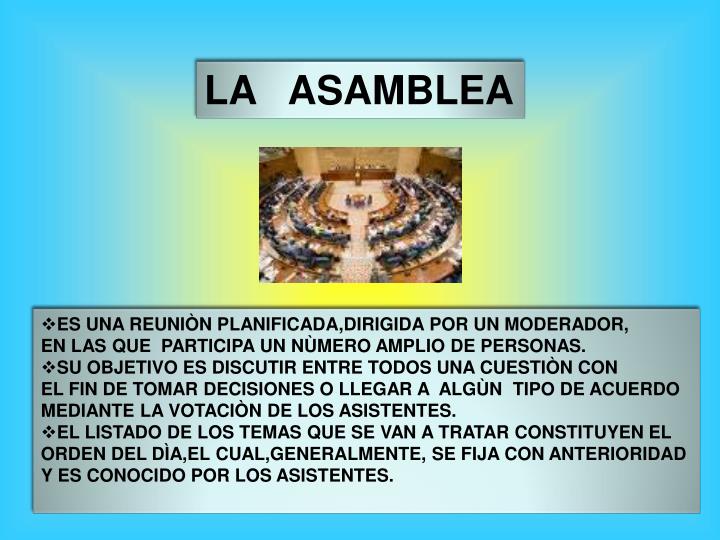The image depicts an assembly, likely a political or governing body meeting, set against a bright blue background reminiscent of the sky. At the top, in large black capital letters, it reads "LA ASAMBLEA," suggesting the assembly as the main focus. Below the title, there is a small, somewhat blurry photograph showing people seated in curved rows, possibly facing a central speaker or panel, characteristic of a bureaucratic or courthouse setting. The image emits a yellow light that extends into the photo, adding to its prominence. Underneath the photo, there's a light gray text box containing several bullet points in Spanish, explaining the nature of the assembly. These points describe the planned nature of the meeting, moderated discussions, the objective of decision-making through attendee voting, and a predetermined agenda known to all participants.